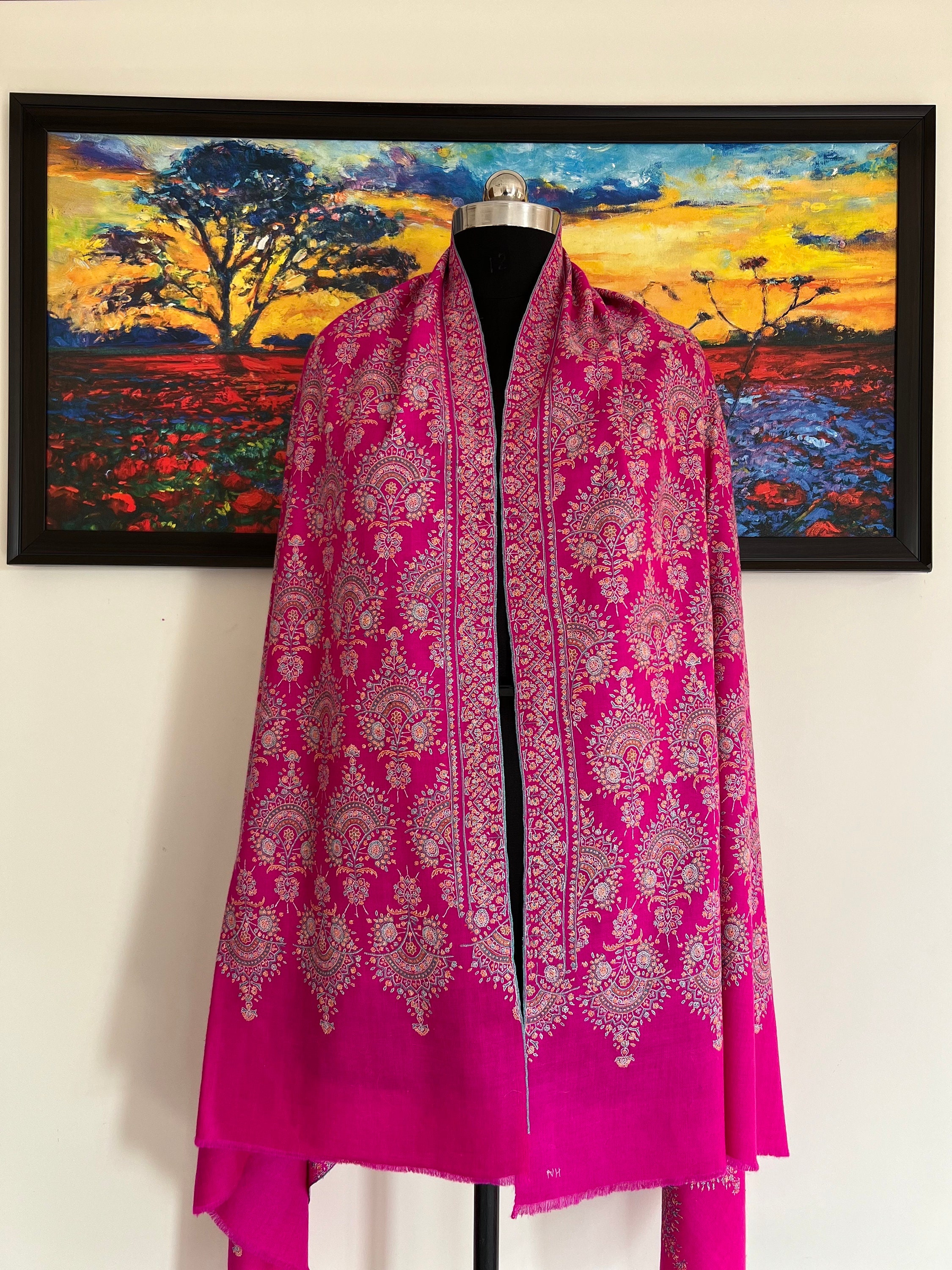This image captures a vibrant indoor scene featuring an intricately designed shawl displayed on a sleek black mannequin torso. The shawl, which might also be a pashmina or wrap, is an eye-catching magenta, almost hot pink, adorned with complex diamond patterns that are composed of myriad small, colorful circles. These diamond motifs are spaced just enough to create an illusion of magenta lines running through them. The intricate patterns include hues like green, blue, red, and orange, contributing to its fractal-like, possibly Asian-inspired design.

The mannequin has a distinctive golden cylindrical cap with an additional golden attachment, adding a touch of elegance. This setup stands against a pale yellow or white wall, which is adorned with a striking oil painting. The painting, framed in black, depicts an abstract landscape rich in color, featuring red flowers, green fields, and a small body of water. The scenery includes trees, primarily on the left side, with another smaller tree on the right, partially hidden by the shawl. The sky in the painting transitions from a vibrant yellow with blue clouds above to more conventional blue tones, suggesting a scene bathed in golden sunlight.